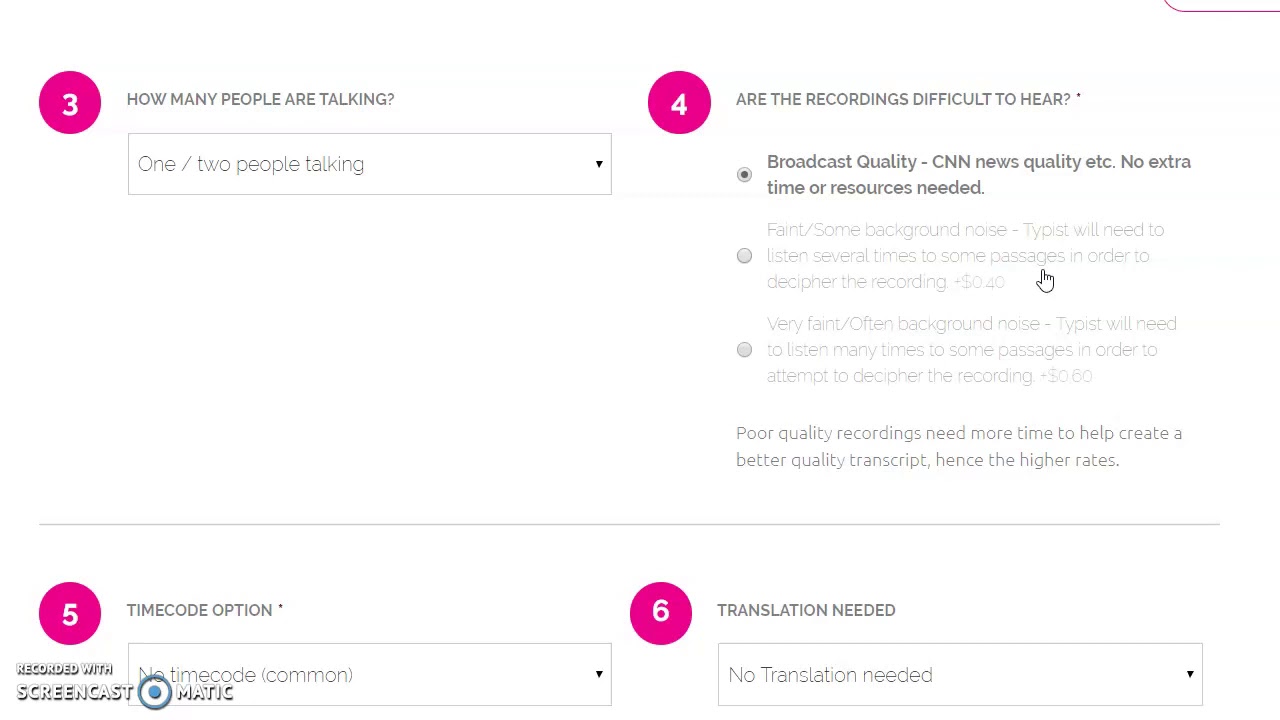This caption appears to describe a process for evaluating and transcribing audio recordings. Below is a more detailed and cleaned-up version of the caption to make it suitable for describing an image representing a transcription setup or workflow:

---

"A transcriptionist is evaluating the quality of an audio recording of one or two people conversing. The recording is of broadcast quality, similar to CNN news quality, requiring no additional time or resources to transcribe. The transcriptionist notes that poor quality recordings would demand more time to produce a high-quality transcript. The recording was made using Screencast-O-Matic and does not include a timecode, which is common for such tools. No translation is necessary for this task."

---

This version is more descriptive and organized, providing clear context about the transcription process, the quality of the recordings, the tools used, and the need for translation.